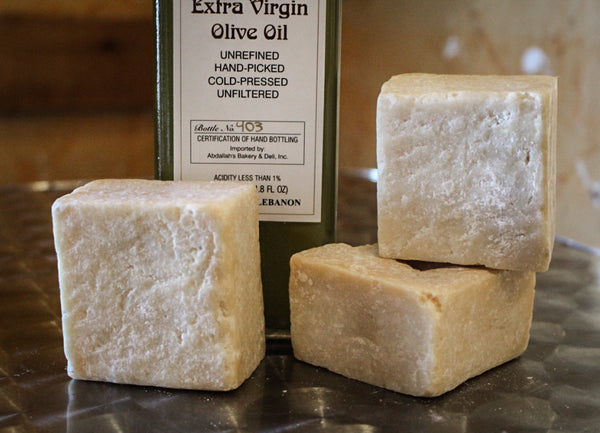The image depicts a photograph taken indoors on a shiny, stainless steel table. On the left side of the table sits a green bottle with a white label featuring black text. The label reads: "Extra Virgin Olive Oil, Unrefined, Hand-Picked, Cold-Pressed, Unfiltered, Bottle No. 403, Certification of Hand Bottling, Imported by [Bakery’s Name], Lebanon." The handwritten "403" provides a personal touch representing the bottle number. To the right of the bottle are three perfectly square, white blocks, which seem to resemble cheese with a crumbly surface texture, though there's speculation they could be soap. The background consists of neutral brown and beige tones, emphasizing the main objects in the foreground.